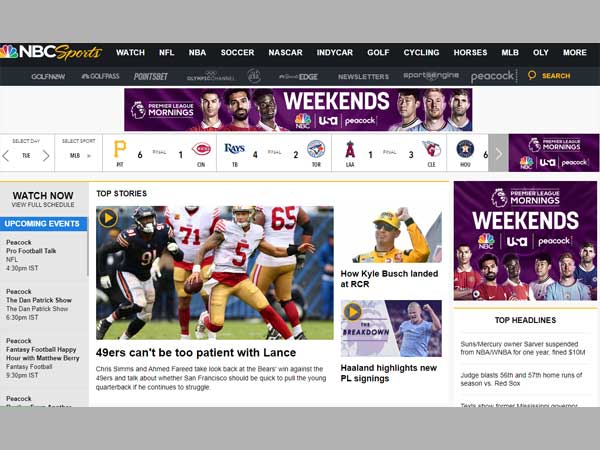This is a detailed description of a webpage from the NBC Sports website:

The webpage features the NBC Sports logo prominently on the left side, displaying a colorful peacock with feathers in yellow, orange, red, purple, blue, and green. The word "NBC" appears in white, while "Sports" is written in yellow. 

Below the logo, a navigation bar presents options such as "Watch NFL," "NBA," "Soccer," "NASCAR," "IndyCar," "Golf," "Cycling," "Horses," "OLY," and more. 

A secondary navigation strip follows with links labeled "Golf News," "GolfPass," "PointsBet," "Edge," "Newsletter," and "Peacock", alongside a search icon.

An advertisement banner below the navigation bars highlights "Premier League Mornings" on weekends, featuring the Peacock streaming service.

Further down, the page displays various sports games and their respective scores, followed by a section labeled "Top Stories." 

Key headlines include:
- "49ers Can't Be Too Patient with Lance"
- "How Kyle Busch Landed at RCR"
- "Highlights New PL Signings"
- "Weekend Premier League Mornings: Weekends on USA and Peacock"

The webpage is a comprehensive hub for sports news, live streams, and scores, organized for easy navigation and accessibility.